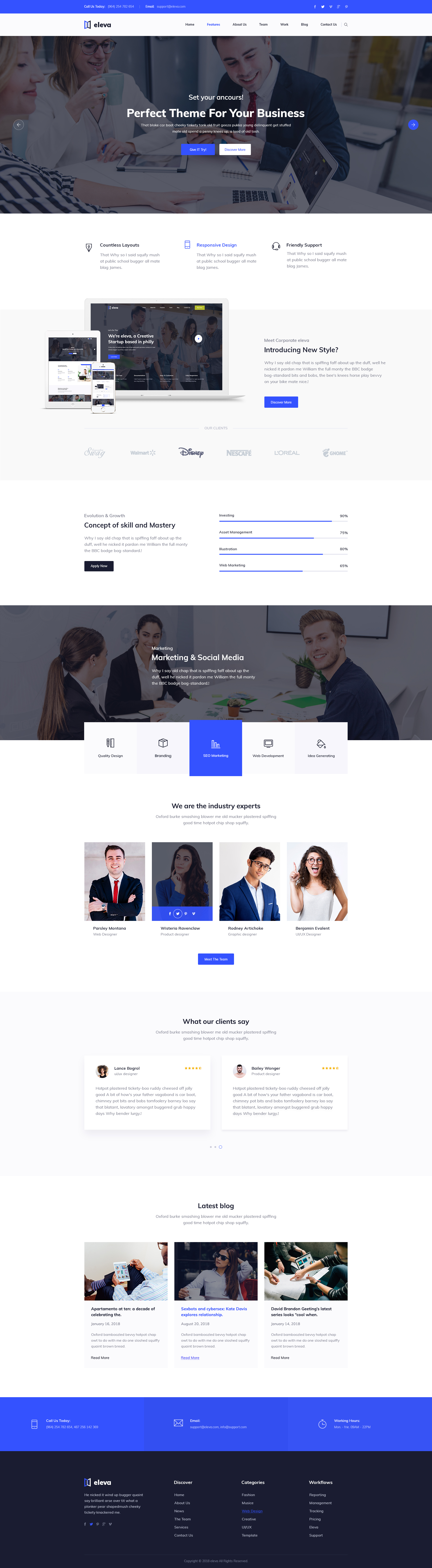A screenshot from the Eleva website showcases various sections meant to highlight its business theme features. The top section prominently displays the tagline, "Perfect Theme for Your Business. Set Your Own Course," against a background where two women and a man are gathered around a laptop, all smiling. 

Below this, a section introduces a new style, though the accompanying text is slightly blurred. To the left of this section, there are images of a laptop, an iPad, and an iPhone. Directly beneath, another blurred section reads, "Concept of Skill and Mastery," accompanied by graphs and percentages that are too obscured to decipher.

The next visible area is a long gray rectangle proclaiming "Marketing and Social Media," featuring a slightly grayed-out photo of three people: two women on the left and a man on the right. This section is followed by a caption listing services such as Quality Design, Branding, Marketing, Development, and Idea Generation, with a statement beneath that reads, "We are the industry experts."

The final part of the screenshot shows a group photo of four people—two men and two women—but their names remain unreadable due to the image being out of focus.